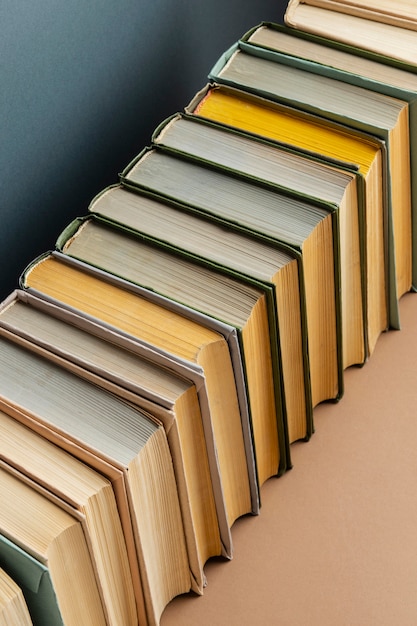In this indoor image, the background features a bluish wall in the upper left corner and a peach-colored shelf or table in the bottom right corner, forming a distinctive diagonal division. Between these contrasting backgrounds, there is a neatly arranged row of hardback books. The books are stacked with their bindings facing the blue wall and their pages exposed towards the peach shelf. The collection includes books of various sizes, showcasing predominantly white pages, with one book notably having bright yellow edges. Altogether, there are at least fifteen books in the stack. The books are organized on a brown table, with their covers partially visible, adding to the intricate details of this visually appealing arrangement.